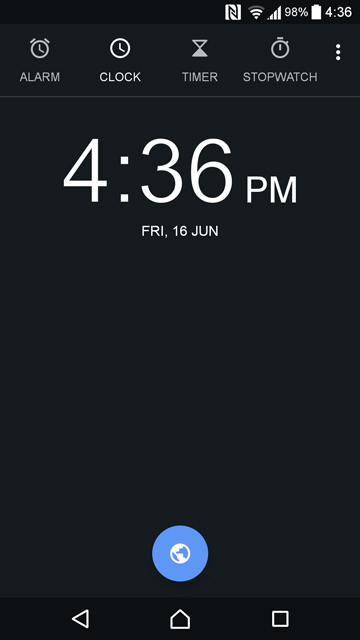This image is a screenshot of a smartphone displaying a black background. At the very top right of the screen, there are several status icons, including a Wi-Fi signal, cellular signal bars, a battery percentage reading "98%", a full battery icon, and the time "4:36". Directly beneath this, there is a larger banner area featuring four symbols: a clock icon labeled "Alarm", another clock icon labeled "Clock", a timer icon labeled "Timer", and a stopwatch icon labeled "Stopwatch". 

The majority of the screen is blank and black, with the current time "4:36 p.m." prominently displayed in large white letters in the upper middle section of the screen. Below the time, in smaller white letters, the date is displayed as "Fri, 16 June". At the very bottom of the screen, there are three navigation icons in blue: a left-facing triangle for "Back" on the bottom left, a circle for "Home" in the center, and a square for "Recent Apps" on the bottom right.